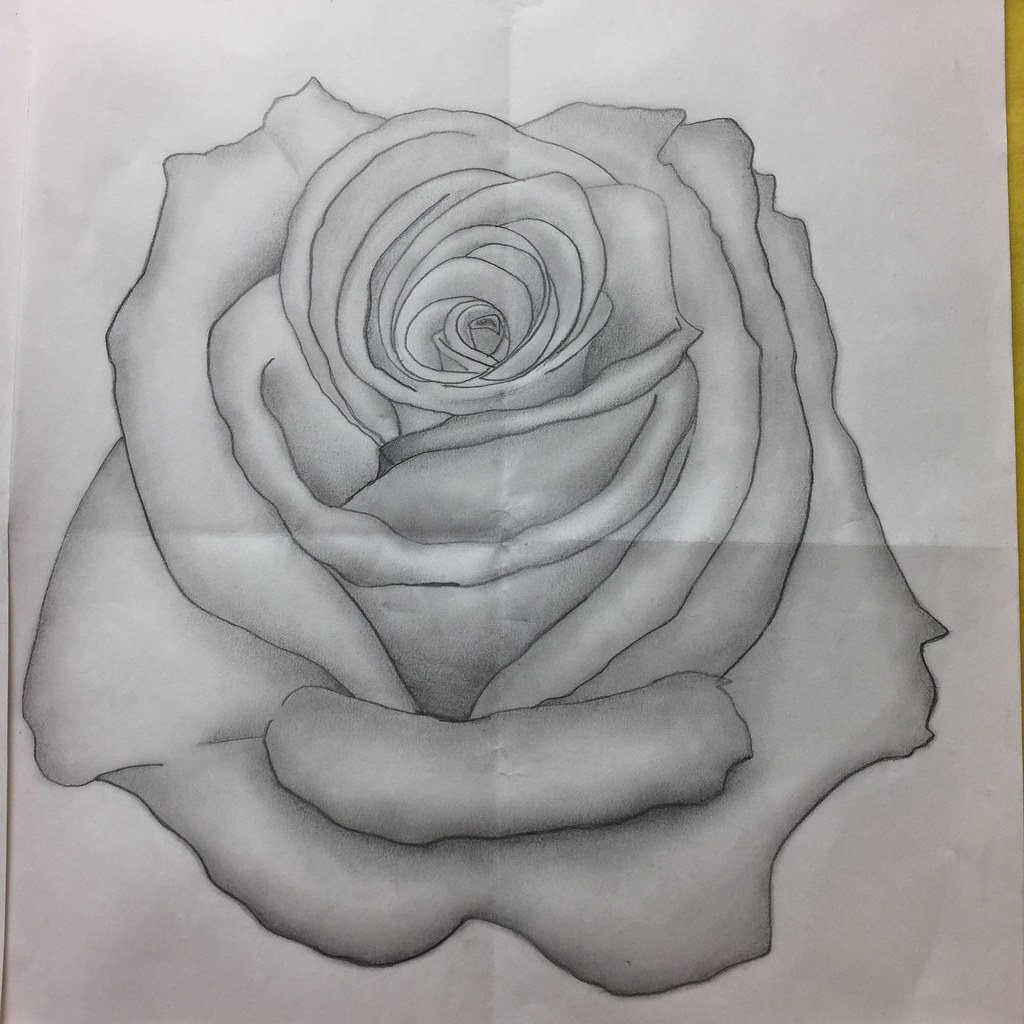This image features a detailed black-and-white pencil drawing of a rose on a white, rectangular piece of paper. The rose is outlined in dark black pencil, with intricate shading that enhances the depth and texture of each petal. The outer petals are delicately folded outward, while the inner petals remain tightly swirled, suggesting the rose is not fully open. The paper itself shows four fold lines extending from the center to each edge—top, bottom, right, and left. Additionally, a hint of a green surface is visible at the top right corner of the composition, adding a subtle touch of color to the otherwise monochrome drawing.